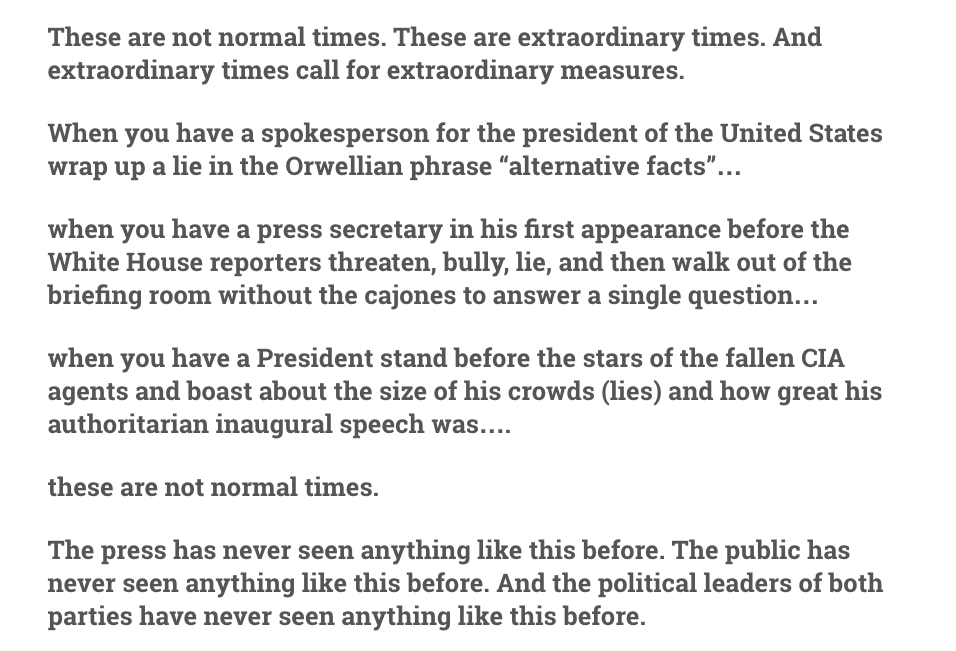The image depicts a typed paragraph displayed on a computer screen. The white background contrasts sharply with the black text, making the words stand out.

The text begins emphatically with the phrase: "These are not normal times, these are extraordinary times. And extraordinary times call for extraordinary measures." It then transitions into critical commentary, stating:

"When you have a spokesperson for the President of the United States wrap up a lie in the Orwellian phrase, 'alternative facts'... 

When you have a press secretary in his first appearance before the White House reporters threaten, bully, lie, and then walk out of the briefing room without the conjoins to answer a single question... 

When you have a President stand before the stars of the fallen CIA agents and boast about the size of his crowds (lies) and how great his authoritative inaugural speech was... 

These are not normal times.

The press has never seen anything like this before. The public has never seen anything like this before. And the political leaders of both parties have never seen anything like this before."

The stark format, with ample spacing between the paragraphs, emphasizes the gravity and unprecedented nature of the circumstances being described.